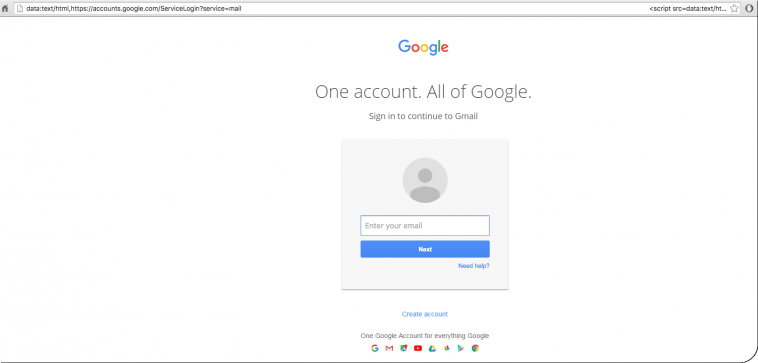A screenshot of a computer screen displaying the Google login page. At the top, there is a web address bar that reads "data:text/html, https://accounts.google.com/service/login/service=mail." To the left of the address bar, there is a home button icon. 

Centrally located on the page is the prominent Google logo. Below the logo, text reads "One account. All of Google. Sign in to continue to Gmail." 

Within a central login box, there is a gray profile icon, beneath which is a text field labeled "Enter your email." Directly below this text box is a blue button with white text that reads "Next." To the bottom right of this button is a hyperlink text that says "Need help?"

Outside the login box, at the bottom center of the screen, is a "Create account" option. Below this, the text reads "One Google account for everything." Beneath this text, there is a row of various symbols representing different Google services and features.